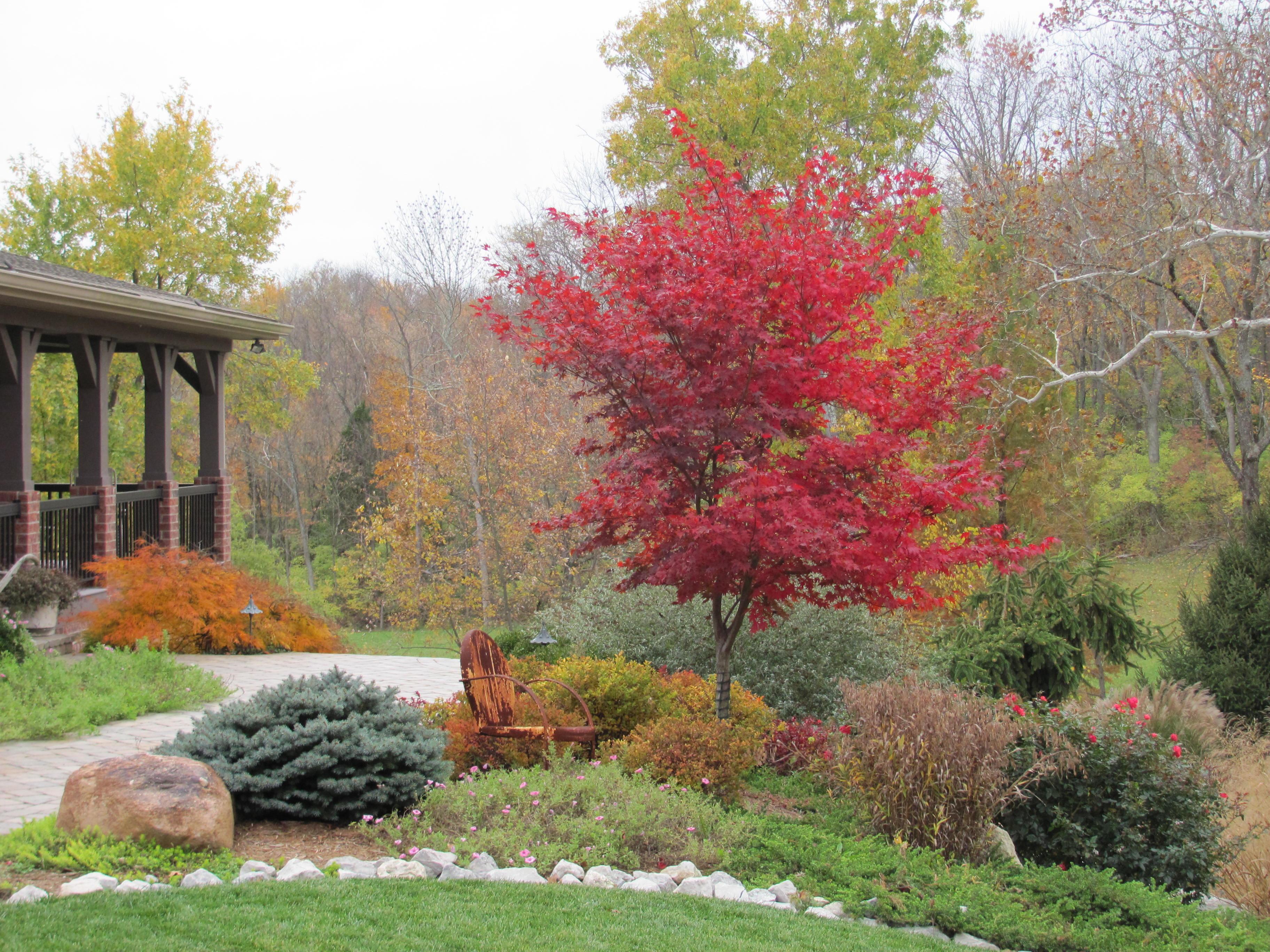This autumn photograph captures a picturesque front yard scene. The vibrant centerpiece is a large, bright red-leafed tree that dominates the middle of the frame. Surrounding this tree are a variety of bushes and smaller shrubs in hues of green, pink, and orange, some of which are adorned with delicate, pink flowers. At the base of this rich foliage, the green grass is neatly outlined by a line of gray and white rocks, which includes a prominent brown boulder partially covered with moss. Adjacent to this rocky setup, there is an old, weathered wooden rocking chair, suggesting a cozy spot to enjoy the fall scenery.

To the left, a brick pathway, wet and shiny, curves gently off towards a gazebo, which features a sturdy brick base with decorative metal railings between brick pillars, each topped with wooden supports for the roof. The pathway hints at leading to a porch or enclosed area, characterized by vertical posts and railings.

In the background, a blend of yellowing and bare trees, as well as trees with orange leaves, stretch across a landscape of gentle hills, creating a rich tapestry of autumn colors. The sky above is an overcast white, completing the serene fall atmosphere of the scene.